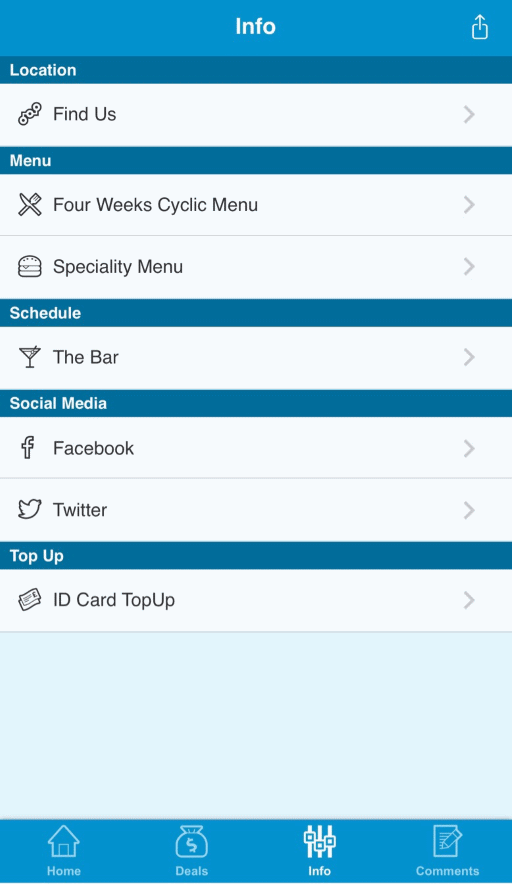The image is a screenshot of a smartphone application in a vertical (portrait) orientation. At the top of the screen, there's a blue bar with white lettering that reads "Info." To the right of this text is a square icon with rounded corners featuring an upward-pointing arrow.

The bottom section of the screen displays a navigation bar with several icons and corresponding labels. From left to right, the icons are:

1. A home symbol with the word "Home" below it.
2. A money bag icon displaying a dollar symbol, with "Deals" underneath.
3. An icon of vertical lines with squares on them, labeled "Info."
4. An icon resembling a piece of paper with horizontal lines and a slanted pencil, labeled "Comments."

The main body of the app contains different sections, each with its own icon and label:

1. **Location:** Accompanied by a symbol and the text "Find Us."
2. **Menu:** Contains two sub-options:
   - "Psilic Menu" (possibly misspelled or unclear)
   - "Specialty Menu"
3. **Schedule:** This section has an icon shaped like a bar.
4. **Social Media:** Consists of two items:
   - The Facebook icon with the text "Facebook"
   - The Twitter icon with the text "Twitter"
5. **Top Up:** Displays an icon on the left and to its right "ID Card Top-Up."

The area towards the bottom of the app has a light teal background color, which transitions into the bottom navigation bar mentioned earlier.